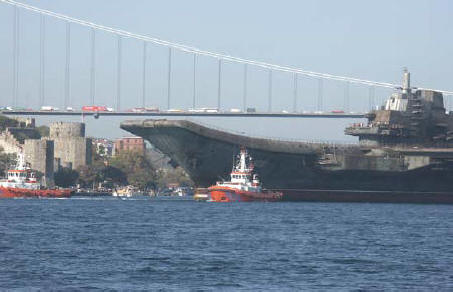The photograph captures a bustling daytime scene of an expansive waterway with deep blue ocean water near the foreground. Dominating the center of the image is a small orange and white tugboat, positioned against the backdrop of a massive dark gray warship extending to the right side of the frame. To the far left, another orange and white tugboat is situated closer to the shore. The distant shore is adorned with a cascade of gray cement structures resembling castles climbing up a hillside, hinting at a fortified or historical area. The shore also features a square red brick building, shrubs, trees, and a cement wall.

Above this maritime scene, a sprawling suspension bridge spans from one side of the image to the other, its deck crowded with cars and trucks traversing the waterway. The serene blue sky crowns the entire scene, providing a calm background to the lively and complex elements of the photograph. In the far distance, another small white boat can be seen navigating the waterway, adding depth to the vivid and detailed portrayal of a waterside location filled with maritime activity and grand architectural structures.